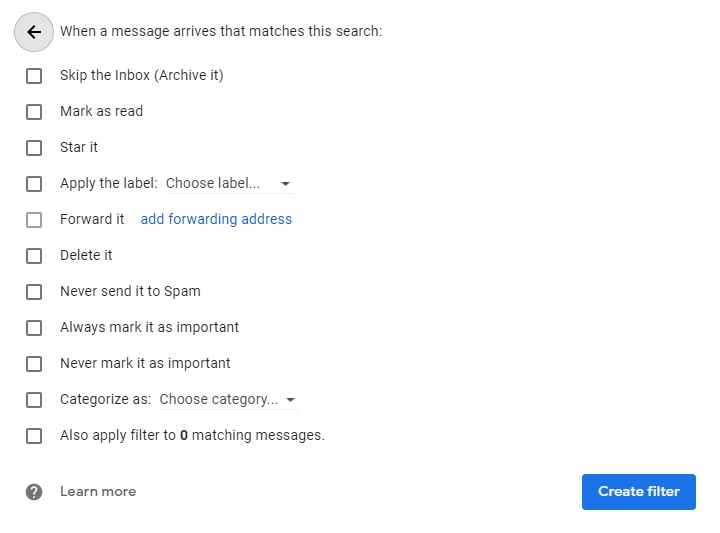The image depicts an email filter settings interface. In the top-left corner, there is a prominent grey circle with a question mark inside, indicating a "Learn More" option. Next to this, a section titled "When a message arrives that matches the search" is visible. Below this, there is a detailed checklist of actions that can be applied to incoming messages:

- Skip the inbox
- Archive it
- Mark it as read or starred
- Apply a label from a dropdown menu
- Forward it to an address
- Delete it
- Never send it to spam
- Always mark it as important
- Never mark it as important
- Categorize using a dropdown menu

Additionally, there is an option to also apply the filter to zero matching messages. The background features a blue wall with a grey filtering interface in the middle.